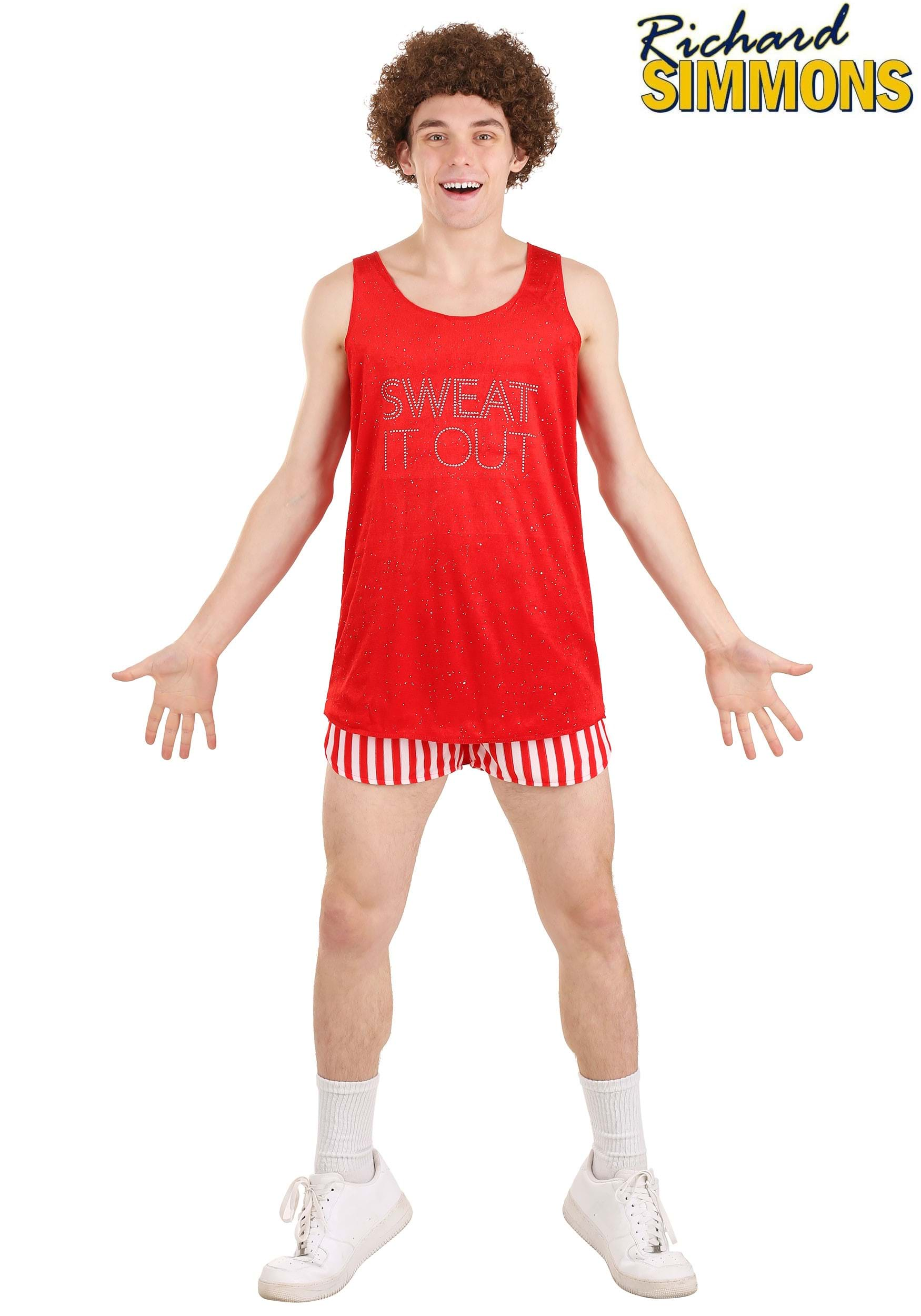The photograph features a young man modeling a Richard Simmons costume in what appears to be a product image, possibly for packaging or a website. The background and flooring have been edited out, leaving the focus solely on the man and his attire against a flat, empty void. The man has a brown curly wig styled in an afro and is smiling with his legs slightly wider than shoulder-width apart. His arms are positioned out from his hips, palms forward with fingers open in a gesture reminiscent of jazz hands. He wears a sleeveless red tank top with "Sweat it Out" written on the front in gray text. His shorts are red and white with vertical stripes, fitting loosely and reaching his mid-calf. Complementing his outfit, he has on white shoes with white laces and tall white socks that rise to his mid-calf. In the top right corner of the image, the name "Richard Simmons" is displayed, with "Richard" in black cursive and "Simmons" in yellow capital letters outlined in black, emphasizing that this is a costume inspired by the celebrity fitness instructor Richard Simmons.